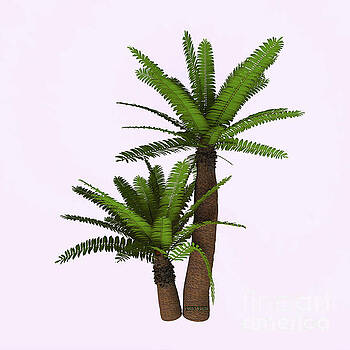The image depicts a computer-generated design featuring two artificial palm trees set against an off-white background with a slight pinkish hue. The palm trees have medium brown trunks and long green fronds clustered at the top. The taller palm tree stands on the right side of the image, while the shorter one is positioned to the left. The shorter tree appears slightly cut off. The background is plain without any specific setting, and there seems to be small, barely legible text at the trunk of the right palm tree, possibly saying "tree." The overall composition suggests the trees are floating in space, without any indication of ground or surroundings.